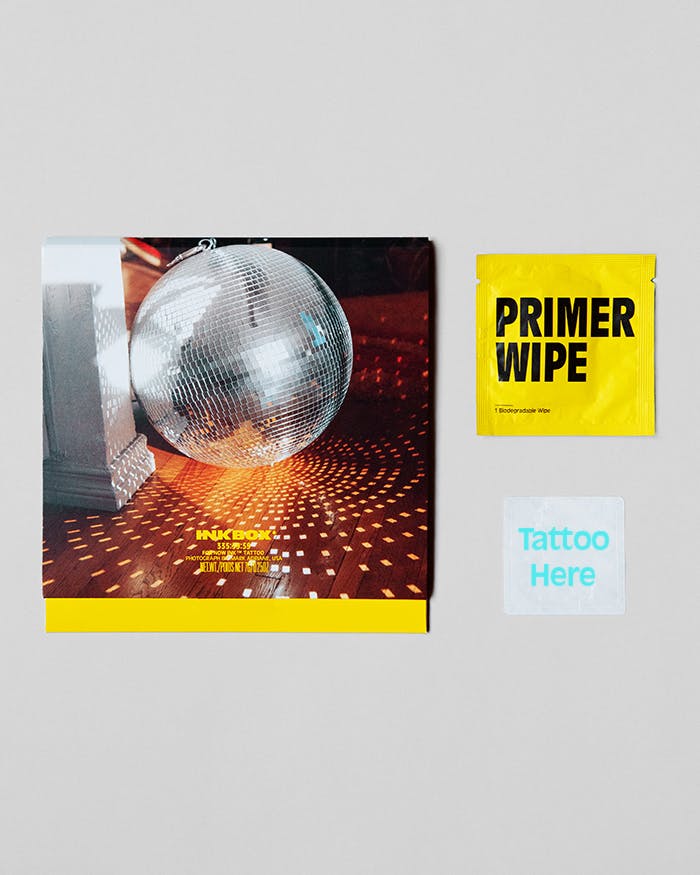The image features a display of three distinct items pinned on an off-white wall. To the left, there's a larger poster showcasing a disco ball on a wooden floor, with its light patterns illuminating the surface. Above the disco ball, the text "INKBOX" is prominently displayed in yellow, with some additional, smaller text below that is not clearly legible. The center of the image features a small yellow square labeled "PRIMER WIPE" in black lettering. To the right, there's a white package with "TATTOO HERE" written in blue letters. The overall arrangement suggests a promotional display, possibly for related products or services, set against a white backdrop, creating a visually cohesive layout.